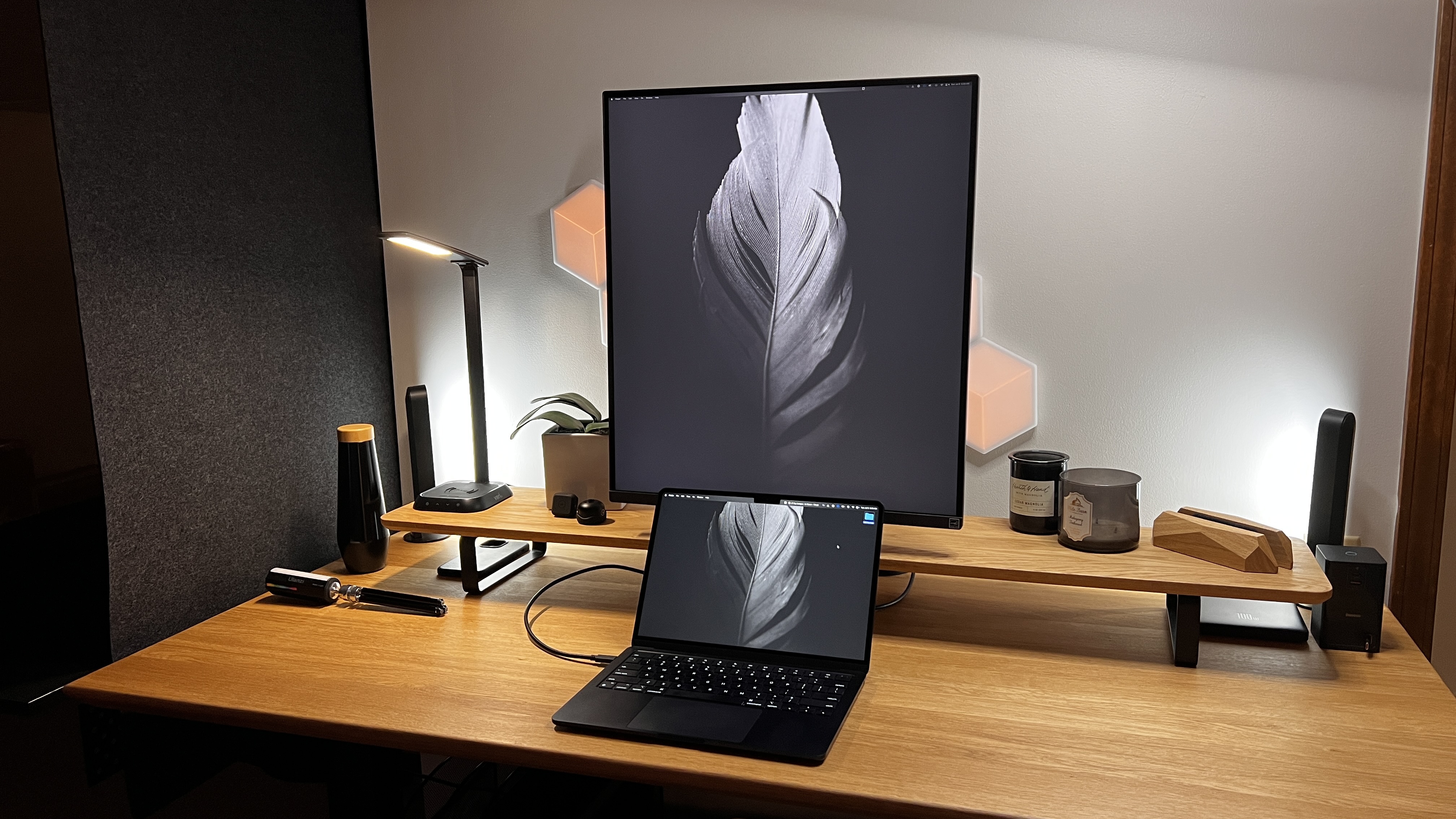This photograph showcases a modern, stylish desk setup featuring a two-level brown desk. Positioned centrally at the lower level is an open laptop, while directly behind it on the higher level stands an unusual, vertically-oriented external monitor. The monitor displays a white feather, and although taller than it is wide, it is not a perfect square and retains an unconventional dimension even when rotated.

To the left of the monitor sits a green plant and a table lamp, adding a touch of nature and ambiance to the workspace. To the right, a collection of jars can be seen, contributing to the organized and functional aesthetic. Additionally, a sleek black water bottle rests on the far left side of the desk, adjacent to the laptop. The back wall features contrasting colors: a gray section to the left and a white section behind the monitor, enhancing the modern decor. Small speakers are placed on the right side of the raised area, completing the setup and adding auditory functionality to the workspace.